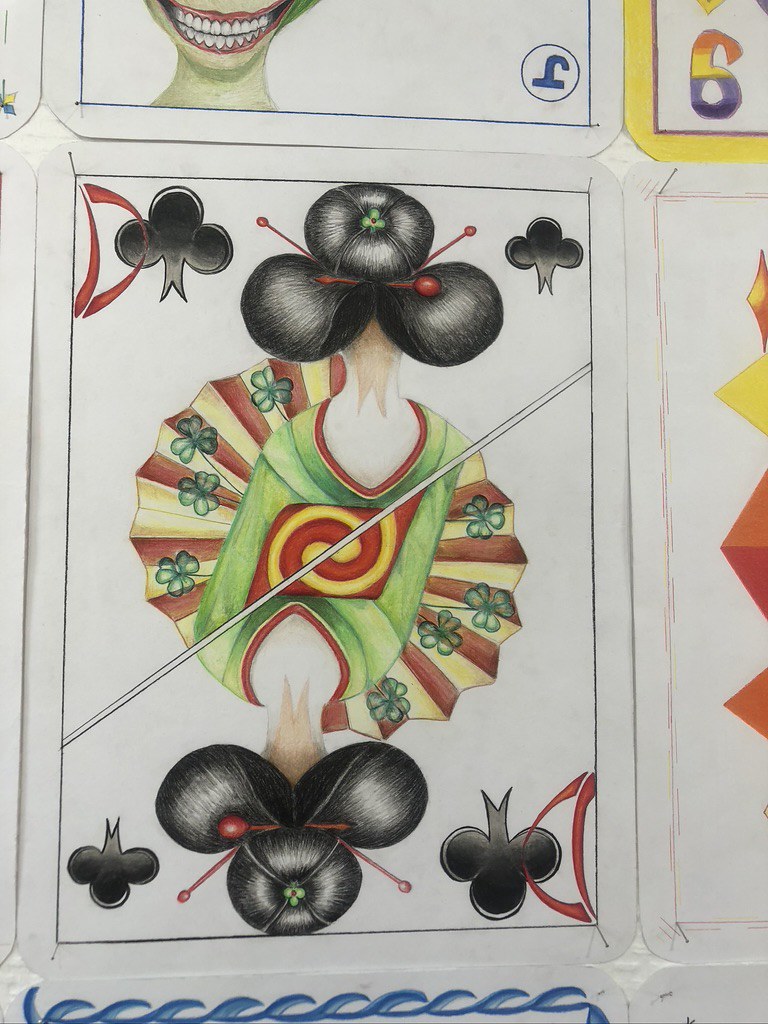The image depicts a collection of eight playing cards, with one card prominently featured in the center. This central card showcases a Japanese-inspired design with detailed artwork. It prominently displays the letter "D" in red in both the upper left and lower right corners, each accompanied by a club symbol in all four corners of the card. The main illustration features a geisha-like woman with jet-black hair styled into three buns, each adorned with red hairpins symbolizing clubs. She is dressed in a traditional green gi with a mesmerizing swirl pattern of red, orange, and yellow in the middle. The geisha holds a fan that mirrors this color scheme with red and yellow stripes and green club symbols. The artwork splits diagonally, creating a symmetrical mirror image. Surrounding the primary card, one can see partial hints of other cards, with one neighboring card featuring a joker design and another showcasing red and yellow hues.